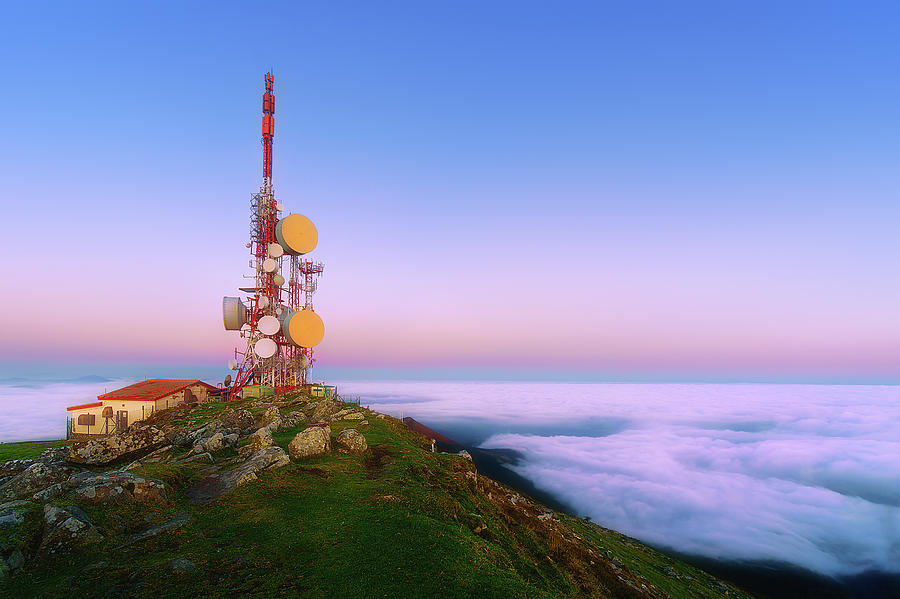A photograph taken outdoors during the daytime captures a scenic shore landscape. The image, rectangular in shape and approximately 6 inches wide by 4 inches high, prominently features a hillside in the lower left corner. This hillside is adorned with large boulders, stones, and patches of green grass. Perched at the top of the hill is a striking white and red building with a red slanted roof, partially obscured by the terrain. Adjacent to this structure is a large metal tower with cylindrical drums, some painted white and others yellow. The lower part of the image is enveloped in low-lying clouds or fog, which melds into a tranquil body of water rendered in shades of blue and white. The sky above transitions through a gradient of colors—from a light blue on the horizon, through purplish-gray, to white, and finally a rich blue at the top. The overall scene exudes a serene and picturesque coastal ambiance.